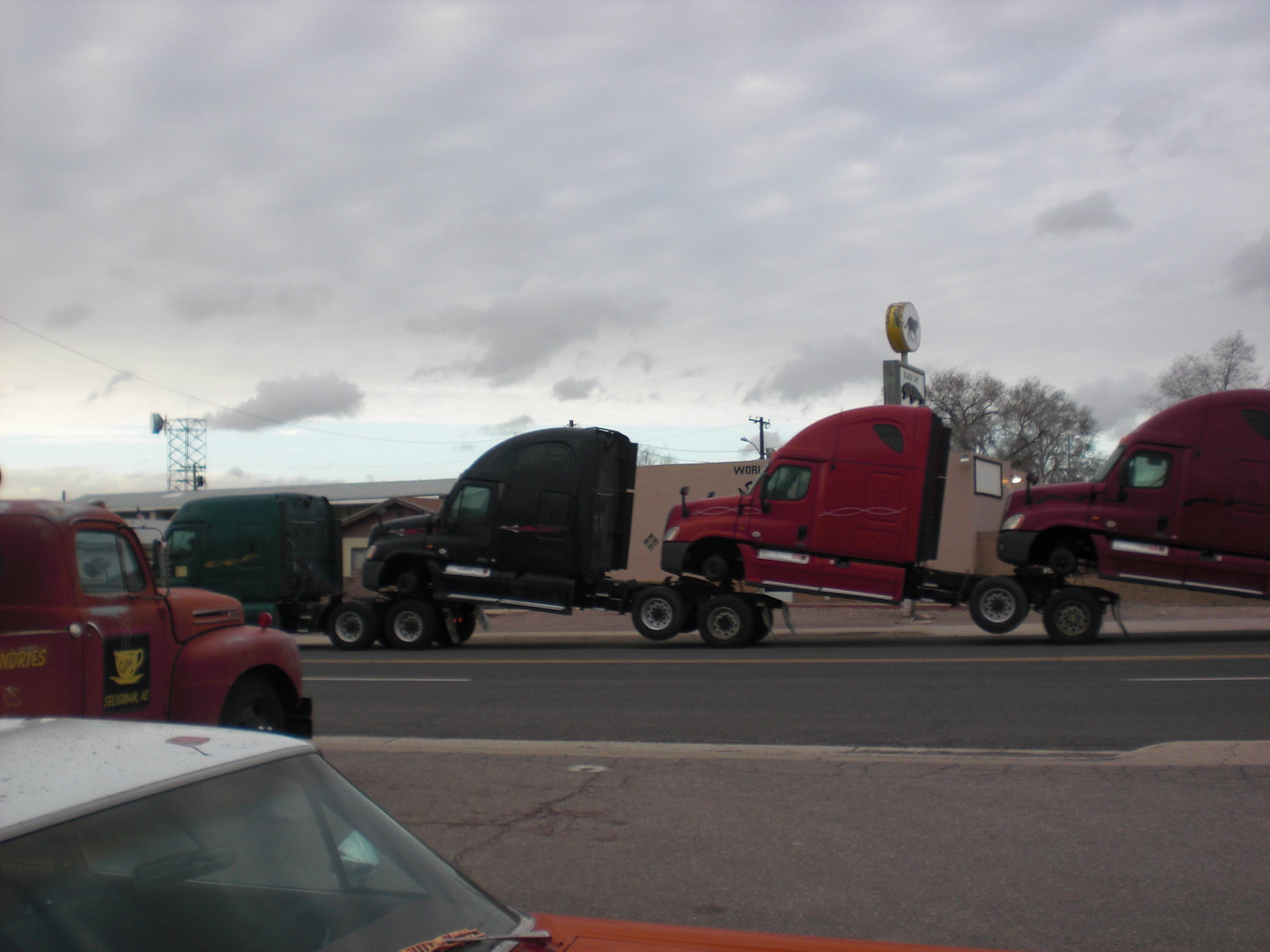Captured from the side of a road or a parking lot adjacent to it, this photograph vividly portrays a line of semi-trucks in an unusual arrangement under a gray, cloud-filled sky. The primary focus is on a leading dark green semi-truck hauling other tractor-trailer cabs stacked in a peculiar manner: the front end of each truck is propped onto the back of the one in front, creating a chain of four trucks. The first towed cab is black, followed by two red cabs, with one appearing burgundy. Notably, these trucks have their front wheels removed to facilitate this configuration, with only their rear tires touching the ground. An old red truck is partially visible on the left edge of the frame, and a building looms indistinctly in the background, adding to the roadside scene's atmosphere.